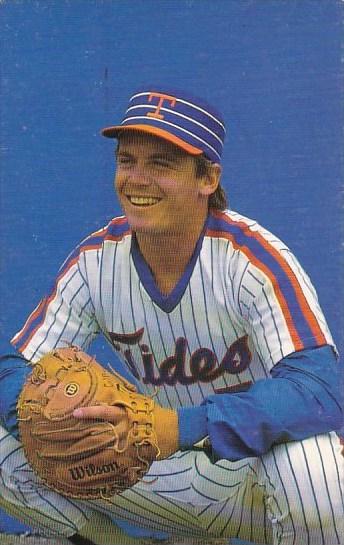This vintage portrait photograph features a Caucasian baseball player, likely from a minor league team, squatting in a classic catcher's stance with his elbows resting on his knees. He is dressed in a distinctive white uniform with blue pinstripes, and his jersey prominently displays the team name "TIDES" in bold blue letters across the front. Over his short-sleeved jersey, he wears a long-sleeved blue shirt that extends to his wrists. His shoulders are accentuated by blue stripes outlined in orange. 

The player is also donning a baseball cap that is blue with white stripes and features an embroidered orange "T" on the front, complemented by an orange bill. He is holding a brown Wilson catcher's mitt, notable for the visible index finger poking through a hole in the mitt. The background is a solid blue, possibly indicative of an outfield backdrop, and adds to the vintage appeal of the photograph. The player is in his 30s, with brown hair and a broad, toothy grin, exuding a sense of joy and pride. The image, captured in a portrait layout, isolates the player as the sole subject, focusing entirely on his cheerful demeanor and distinctive uniform.